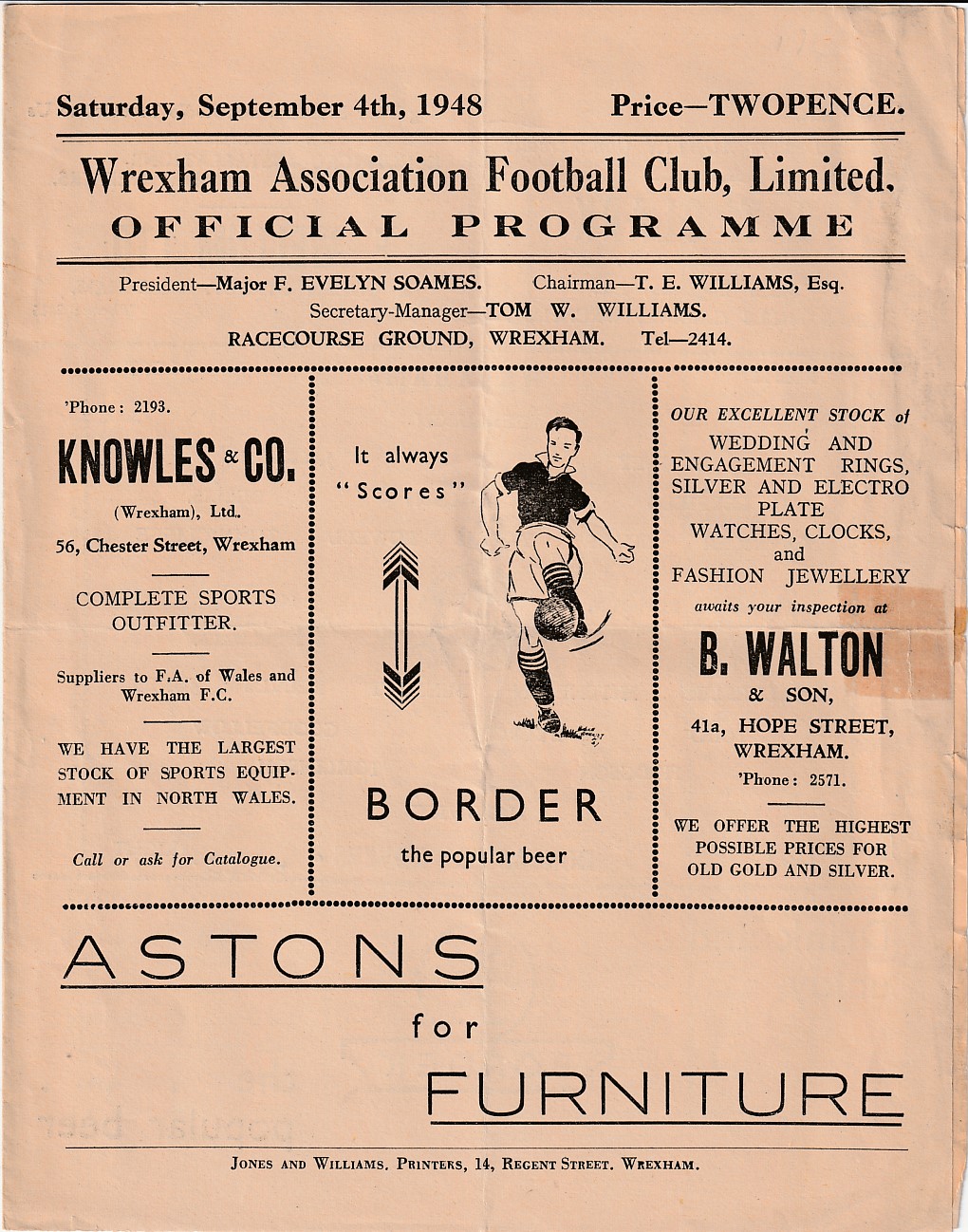This is an image of an old advertisement poster, designed in pink with black text, from the official program dated Saturday, September 4th, 1948, priced at 2 pence. The headline prominently features "Rexham Association Football Club Limited" followed by "Official Program" in all capitals. Below this, it lists the club's officials: President Major F. Evelyn Soames, Chairman T.E. Williams Esquire, and Secretary Manager Tom W. Williams, along with the location "Racecourse Ground, Rexham" and a telephone number "2414."

The poster is divided into three columns of advertisements. On the left, it features Knowles & Company, a complete sports outfitter, claiming to have the largest stock of sports equipment in North Wales, with a call-to-action to request a catalog. In the center, a black-and-white image of a soccer player, dressed in a black jersey and black socks, is captured kicking a ball with his left foot. Adjacent to the player, an advertisement for "Borda, the popular beer" includes the slogan "It Always Scores" with arrows pointing up and down. 

To the right, the ad for B.W. Walton & Son highlights their offerings of wedding and engagement rings, jewelry, watches, clocks, and silver, promising high prices for old gold and silver. At the bottom of the poster, Ashton's for Furniture is prominently featured, and it's followed by a line that credits Jones and Williams Printers, including their address.